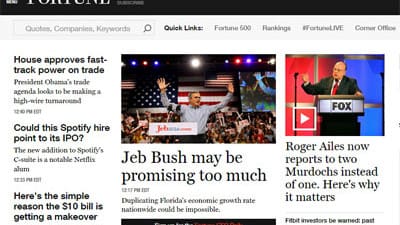The image is a small, panoramic screenshot from a website, presenting a cut-off view of the top section. The visible part includes a long black bar with partially obscured white, all-caps text, likely spelling "FORTUNE." Below this is a gray bar containing a search box with a faint magnifying glass icon and text fields labeled "Quotes," a term starting with 'C,' "Companies," and "Keywords." To the right are quick links with black and gray text, including "FORTUNE 500," "Rankings," and "Featured Live." However, the text is too small to discern completely.

On the left side of the image, there are three article thumbnails with black headlines. The first headline reads, "White House Approves Fast Track Power on Trade," discussing President Obama's trade agenda. The second headline says, "Could This Spotify Hire Point to Its IPO," hinting at significant changes in Spotify's executive team. The third headline is, "Here's the Simple Reason the $10 Bill is Getting a Makeover," though the rest of the article is cut off. Dates and times under each headline are too small to read.

Centrally, a large rectangular image features Jeb Bush with his arms raised and palms outstretched at a rally, wearing a blue shirt. The podium bears the website "jebbush.com" over a white background with red, blue, and orange highlights. Behind Jeb, a crowd is cheering and waving signs, with a giant American flag and two smaller flags flanking Jeb. There’s a screen on the right displaying the same rally scene. The caption below says, "Jeb Bush may be promising too much," followed by a note on the difficulties of replicating Florida's economic growth nationwide. A black bar below the caption is cut off.

To the far right, another image shows a man in a black suit with a red tie, possibly Roger Ailes, at a podium labeled "Fox" on a white background. The microphone has red on the left and blue on the right. Below this image, the caption reads, "Roger Ailes now reports to two Murdoch’s instead of one, here’s why it matters." Beneath is a text box mentioning, "Fitbit investors be warned," but the remaining text is cut off.